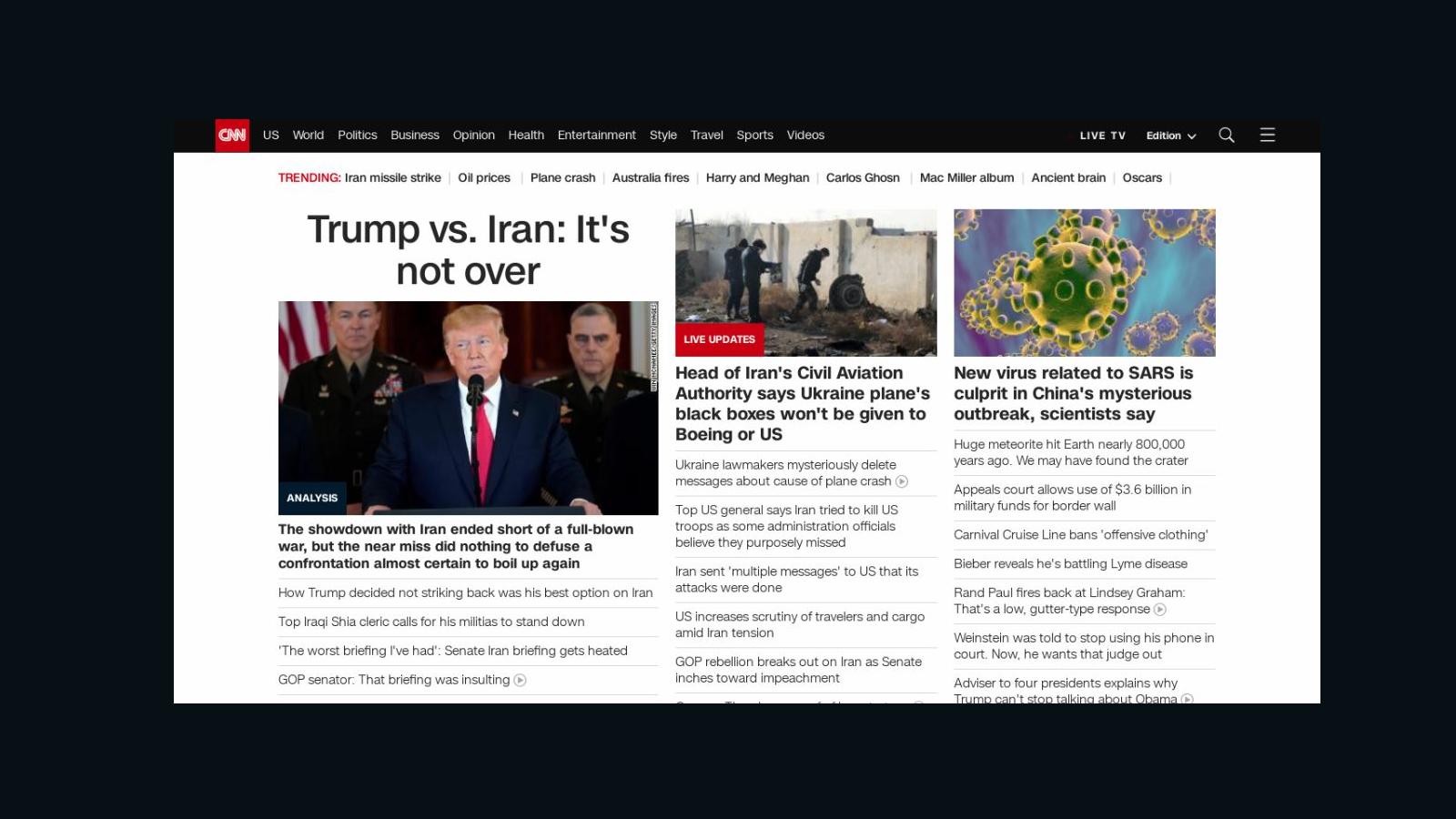An image captures a webpage resembling the CNN homepage, prominently displayed against a solid black background. The page appears to be extracted and pasted onto this backdrop, creating a pronounced thick margin surrounding it. In the top left corner, the iconic CNN logo is highlighted in red. Adjacent to the logo, a series of navigational tabs span horizontally, including categories: US, World, Politics, Business, Opinion, Health, Entertainment, Style, Travel, Sports, and Videos. On the right side, options for Live TV, a dropdown menu labeled "Edition," a search icon, and a triple-line menu symbol are presented in white against the black background.

Beneath the navigation bar, a list of trending topics is displayed in white text. Noteworthy trends include Iran missile strike, oil prices, plane crash, Australia fires, Harry and Meghan, Carlos Ghosn, Mac Miller album, Ancient Brains, and Oscars.

Dominating the page is a headline: "Trump vs. Iran: It's Not Over." The subtext elaborates that while a major conflict with Iran was averted, tensions remain high and likely to resurface. Additional context includes details such as President Trump’s decision to not retaliate militarily against Iran, a call by a top Iraqi Shia cleric for militants to stand down, and reactions from GOP senators describing a Senate-Iran briefing as the "worst briefing" they have experienced.